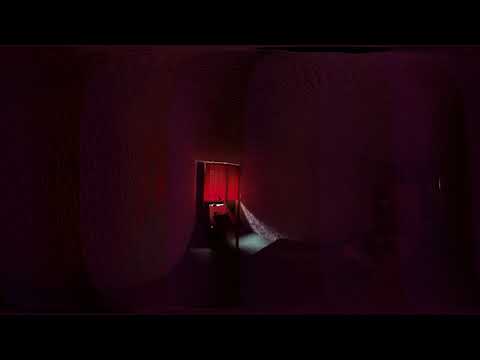The image depicts a dark, indoor setting featuring a variety of unidentifiable objects due to the low lighting. Dominated by a maroon background, the scene is framed by black borders at both the top and bottom. At the center lies a striking red rectangular structure, potentially a window or a banner, surrounded by red curtains. This red element is flanked by shadows and streaks of dark purple and gray, creating a somber ambiance. There is a lighter area below the red rectangle, possibly a light-colored cloth extending towards the lower right, though it does not stretch far. Additionally, there seems to be a curved line emerging from the bottom of the red rectangle, arching towards the lower left. Overall, the setting resembles a narrow corridor or room, with undefined elements casting further ambiguity on the scene.